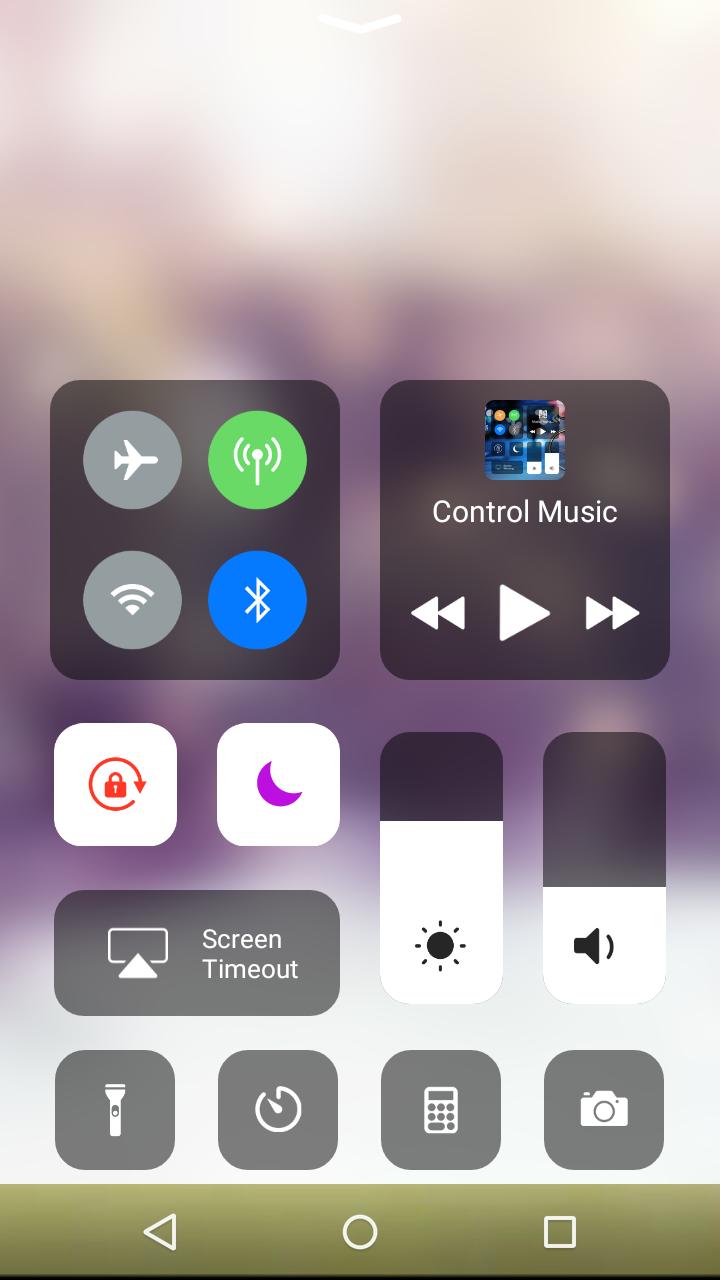The image is a vertically-oriented screenshot taken from an iPhone, depicting the device's control panel. The background is extremely blurred, with only indiscernible colors visible. At the very top center of the screenshot, a downward-pointing arrow icon indicates a swipe-down gesture.

In the center of the image, a gray rectangular box features four circular icons: an airplane, a cell phone signal, Bluetooth, and Wi-Fi. The Bluetooth icon is highlighted in blue, while the cell phone signal icon is illuminated green, signifying active connections.

To the right of this gray box is another section labeled "Control Music," which includes left and right arrow icons for navigation and a central play button.

Below the first gray box, there is a white lock icon with red details. Adjacent to this is a sleep mode icon represented by a purple moon on a white background. Also located in this area is an oblong box for screen timeout settings.

Towards the bottom right of the screen, there are two rectangular sliders: one for brightness and another for sound. The brightness slider is positioned about two-thirds of the way up, indicating a relatively high brightness level, while the sound slider is set approximately one-third of the way up, suggesting a lower volume level.